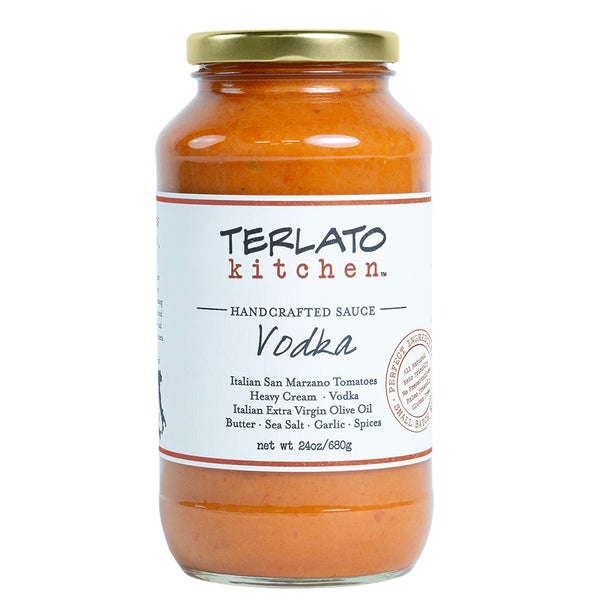The image features a clear glass jar of Terraloto Kitchen Handcrafted Vodka Sauce, prominently set against a clean white background. The jar holds 24 ounces (680 grams) of a light orange, creamy tomato sauce made with Italian San Marzano tomatoes, heavy cream, vodka, Italian extra virgin olive oil, butter, sea salt, garlic, and various spices. The jar is topped with a golden lid. Its simple, paper label is white with black text and is bordered by a delicate red line at the top and bottom. The label also includes a certification stamp of approval, signifying the premium quality of the ingredients. The text on the label highlights the artisan nature of the sauce and offers an overview of its rich, authentic Italian ingredients.